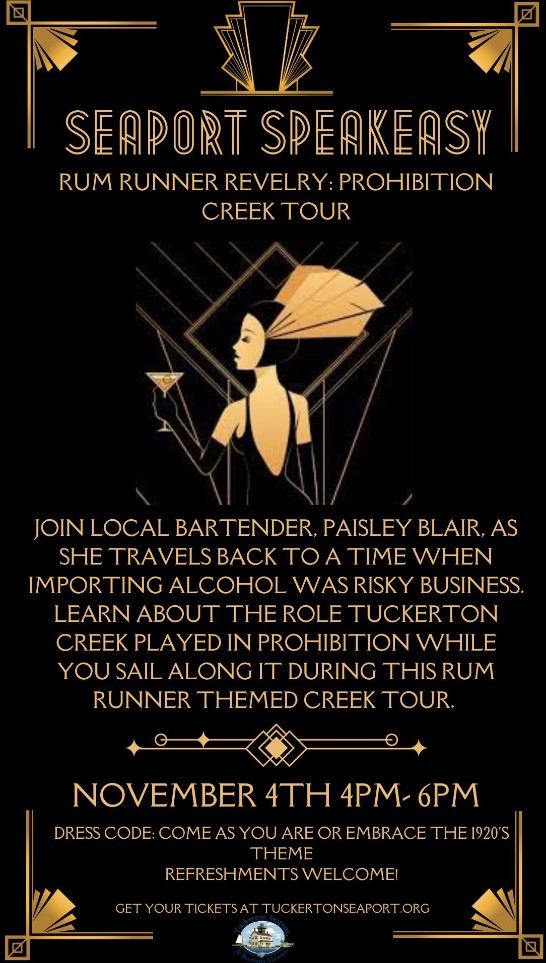This image is a vividly detailed poster for an event named "Seaport Speakeasy: Rum Runner Revelry - Prohibition Creek Tour," set against a black background. The title, written in an elegant Art Deco font, adorns the upper left and right corners, accompanied by intricate gold fan designs also in the corners. At the center is a striking illustration of a woman in 1920s attire, exuding glamour with black hair adorned by a feathered headpiece, and a sophisticated black dress with revealing cutouts. She holds a martini glass with a yellowish drink, her back partially turned, emphasizing the era's style.

Below the illustration, the poster invites attendees to "Join local bartender Paisley Blair as she travels back to a time when importing alcohol was risky business." It promises an engaging historical journey about Tuckerton Creek's role during Prohibition, experienced while sailing along the creek on a rum runner themed tour. The event is scheduled for November 4th, from 4 PM to 6 PM, with a dress code that encourages participants to "come as you are or embrace the 1920s theme." Refreshments are welcome, and tickets are available at tuckertonseaport.org. The poster's detailed gold decorations, including squares, diagonal lines, and diamond patterns, add to the vintage allure, evoking the opulence of the Roaring Twenties.